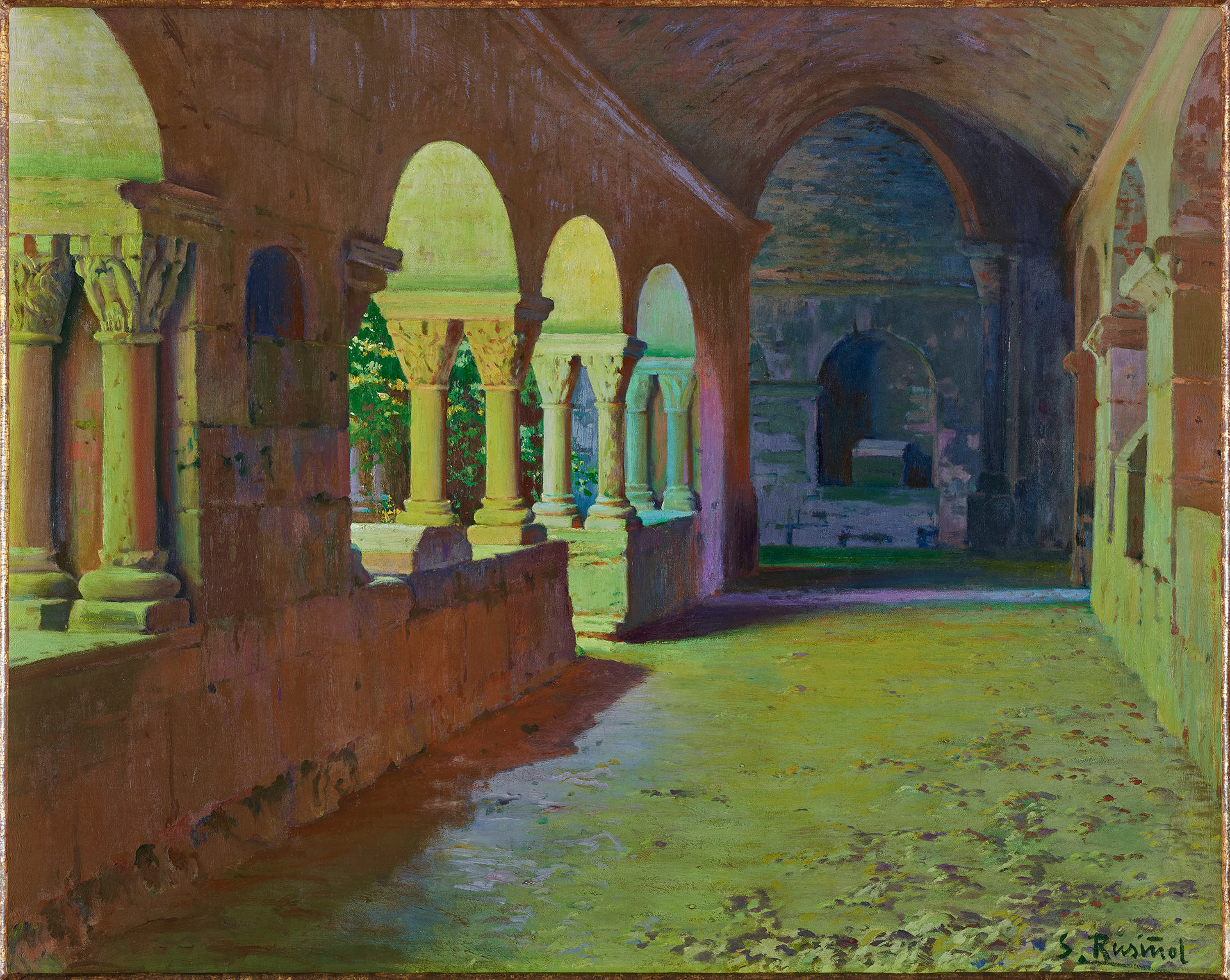This detailed watercolor artwork by S. Roussimol depicts a large, open interior hallway reminiscent of Middle Eastern or Indian architecture, possibly part of a palace or garden-adjacent structure. The scene features multiple high-arching archways supported by weathered stone pillars, creating various pathways through the space. Several archways and cutout windows, sans glass, offer views between sections of the hallway, enhancing the sense of openness. Some arches appear to be decorative niches. 

The ground is rough and dotted with dirt and rocks, while traces of grass and leaves are visible in the background, hinting at outdoor proximity. Light plays a significant role in the painting, casting different hues on the structures; the columns exhibit shades of blue, green, orange, and yellow, suggesting an artistic use of light for effect. The walls and ceiling show a palette of pink, pale turquoise, and other colors that add a slightly whimsical feel to the depiction. Located in the bottom right corner, the artist's signature, "S. Roussimol," is subtly included, with a distinctive horizontal line over the 'M.'